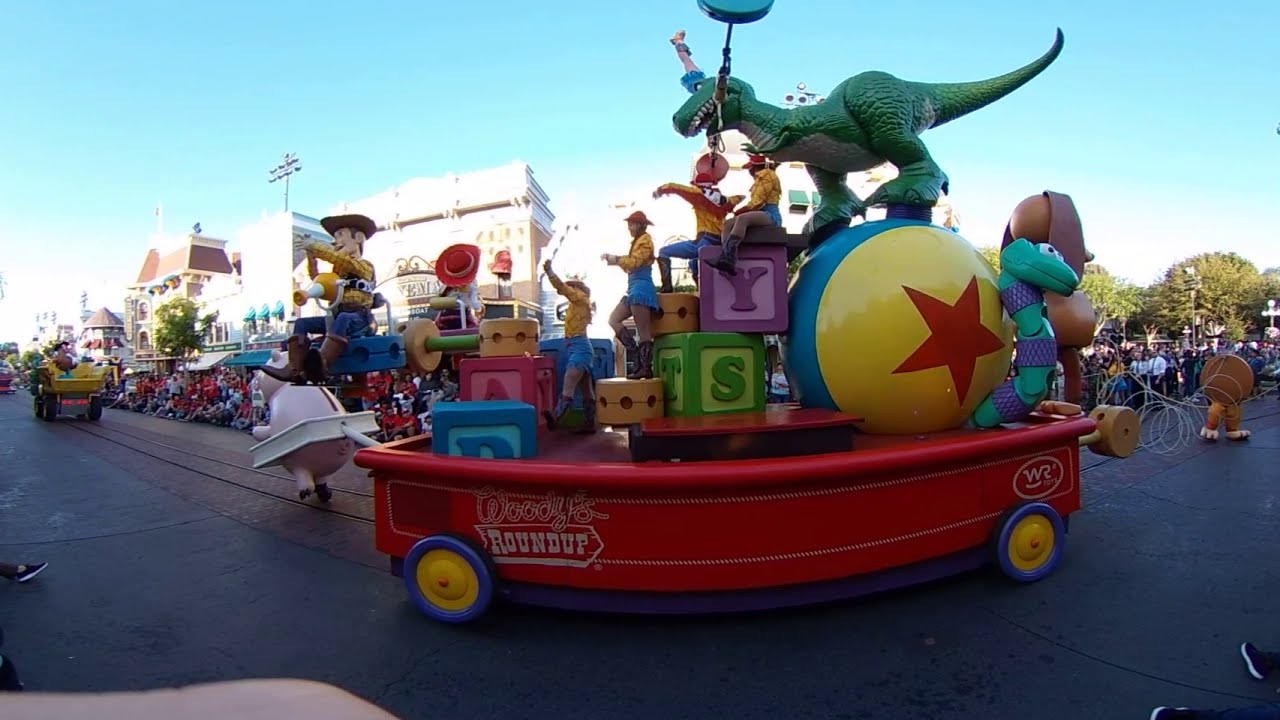In this vibrant outdoor photograph taken during a sunny, cloudless day, we are presented with a lively parade scene. The quintessential feature of the image is a large, eye-catching float in the center, modeled after a red wooden wagon, prominently labeled "Woody's Roundup." This Toy Story-themed float is adorned with an eclectic assortment of oversized toys, including a giant toy dinosaur perched atop a large, half blue and half yellow toy ball with a red star. Surrounding this setup are large toy blocks with visible letters and oversized Tinker Toys. Woody, the iconic character from Toy Story, is seen driving the wagon, which is being pulled by a pig, capturing the whimsical essence of the beloved movie. Additional playful elements include a dog at the back of the float and a snake figurine. The scene is set on a paved road, viewed from the perspective of someone standing among the large crowd gathered to watch the parade. In the background, buildings with classic facades and some trees are visible, enhancing the outdoor setting of this bustling midday event. The photograph bursts with a spectrum of colors including black, gray, tan, red, white, blue, yellow, purple, green, and pink, contributing to the overall festive and joyous atmosphere.